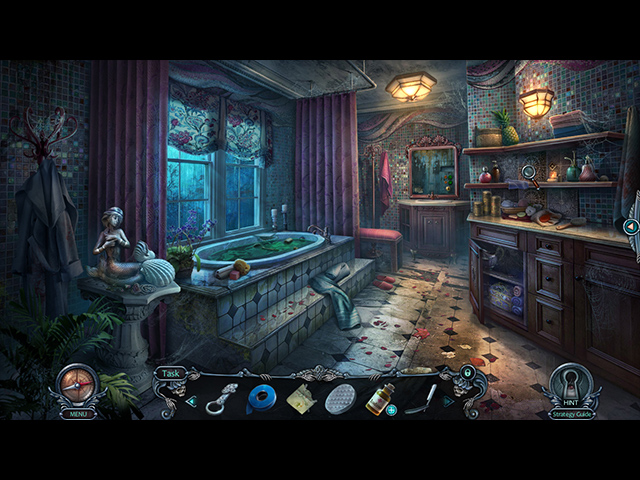The image portrays a luxurious, intricately designed bathroom, resembling a scene from a video game with a slightly mysterious and ancient ambiance. The viewpoint is from atop a vanity table, gazing outward toward the elegant space. Dominating the left side is a majestic marble soaking tub, elevated by a couple of steps and positioned below two ornate curtained windows. Adjacent to the tub stands a sculpted fountain-like statue, adding to the room's antique charm. The bathroom is illuminated by yellow ceiling fixtures, adding warmth to the bluish-purple backdrop and the stone-tiled floor with its triangular black accents. In the distant background is a sink set against an elaborately decorated wall. To the right, an ornately carved wooden dresser with cabinets and drawers supports a variety of bowls, baskets, and a magnifying glass on its shelves. Additional lighting fixtures hang from the ceiling, further enhancing the room's bright and inviting atmosphere. The bottom portion of the image is framed by a status bar, indicating themes and options typical of a strategy game.